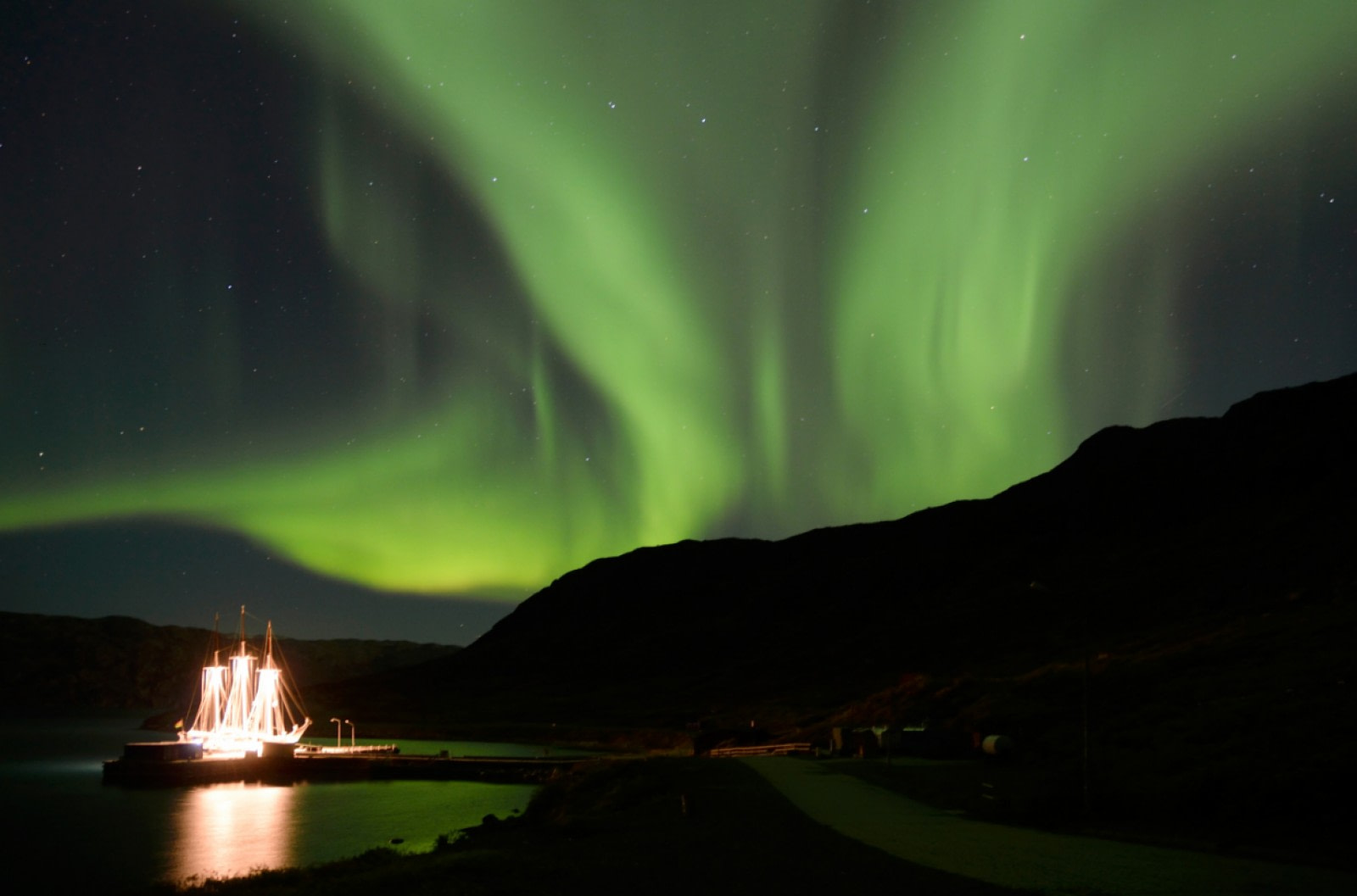This image captures a breathtaking night scene featuring the northern lights, predominantly green with hints of yellow, dancing across a dark and clear sky scattered with stars. The aurora borealis forms undulating waves, with a thicker wave on the right side extending behind a range of dark, bluish mountains. To the left, another green wave curves off upward and leftward, with a slender band in between them. These waves ascend out of the frame, lending a surreal ambiance to the night.

Below the mesmerizing sky, a mountain range can be seen extending across the middle to the right of the image. Dark hills gradually rise from the left to the right side, contributing to the serene landscape. At the base of these hills, on the right, are some buildings and a road emerging from the bottom right corner leading leftward, enhancing the remote, tranquil setting.

In the bottom left corner, the scene shifts to a lakeside with a body of water reflecting the green light from the sky and the white lights from a nearby boat. The boat, gleaming under its lights, is moored near a dock that stretches from the left bottom toward the center. Its reflection ripples across the lake’s surface, adding a dreamy, luminous effect. A sidewalk connects this dock to a small house or structure nearby, completing this captivating nocturnal landscape.